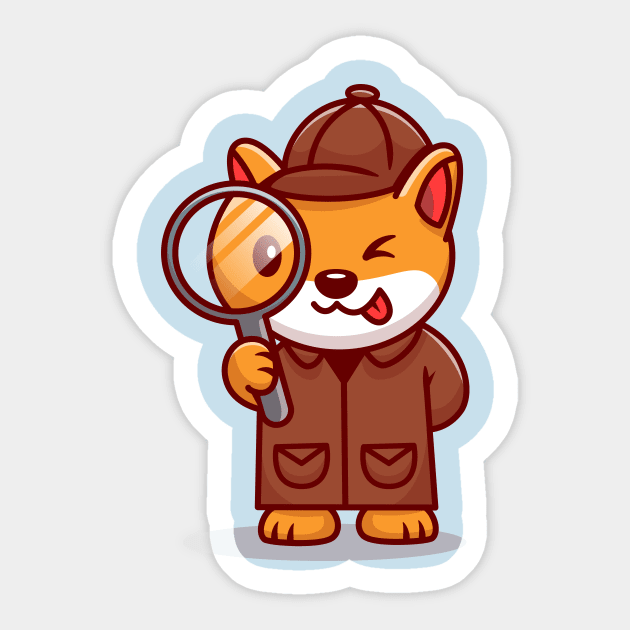This image is a highly detailed, synthesized cartoon of an anthropomorphic orange dog dressed as a detective, reminiscent of Sherlock Holmes. The dog has a white area around its mouth, with its left eye open and its right eye closed, and a red tongue sticking out from the right side of its mouth. It sports a brown detective hat and a long brown trench coat. The dog’s ears are upright with red interiors. The left arm, hidden behind its back, and the right arm holds a gray magnifying glass up to its eye, giving the impression that the dog is scrutinizing the viewer. The image features a light blue background, closely outlined in white to resemble a sticker. The overall background of the image is gray, enhancing the focus on the detective dog character.